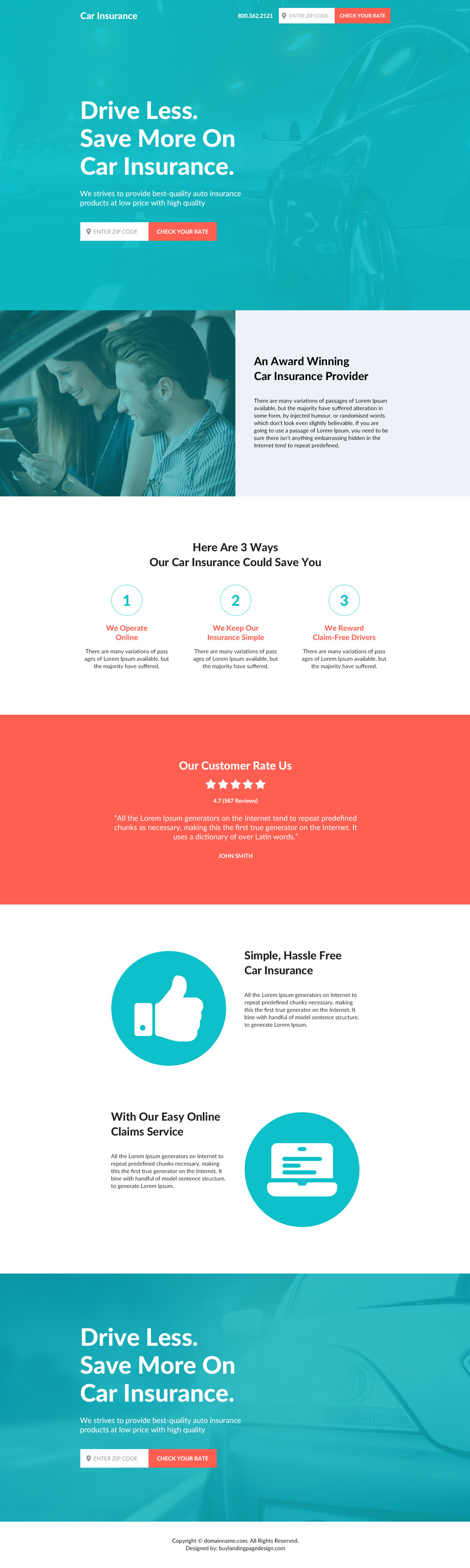The web page appears to be an extended, slightly stretched image of a car insurance provider's landing page. 

At the top, there's a green header area. On the top left corner in white text, it says "Car Insurance," and to the right, there's a phone number along with a white search bar, adjacent to an orange search button. 

Below this, a prominent tagline in big white text reads, "Drive Less, Save More on Car Insurance," accompanied by a line of smaller text beneath it. However, this smaller text is difficult to read due to its size. 

Embedded within a white box, there is a field labeled "Enter a Zip Code," next to an orange button that presumably says "Check Your Rate." 

The background features a green-tinted image of a car. Following this section, it describes the company as an "Award-Winning Car Insurance Provider," accompanied by some additional text. On the left, there is a picture of a man and a woman sitting in a car.

Further down is a section titled "Here are Three Ways Our Car Insurance Could Save You," outlining three benefits in order. Each benefit is highlighted in orange text with additional details in black text underneath. 

Next, there's an orange area with the text "Our Customers Rate Us Five Stars," followed by more accompanying text. Below this, the page emphasizes "Simple, Hassle-Free Car Insurance," highlighting features like "Our Easy Online Claim Service," each supported by brief descriptions.

Finally, the page reiterates the slogan "Drive Less, Save More on Car Insurance," and again displays the zip code entry box with the orange "Check Your Rate" button.